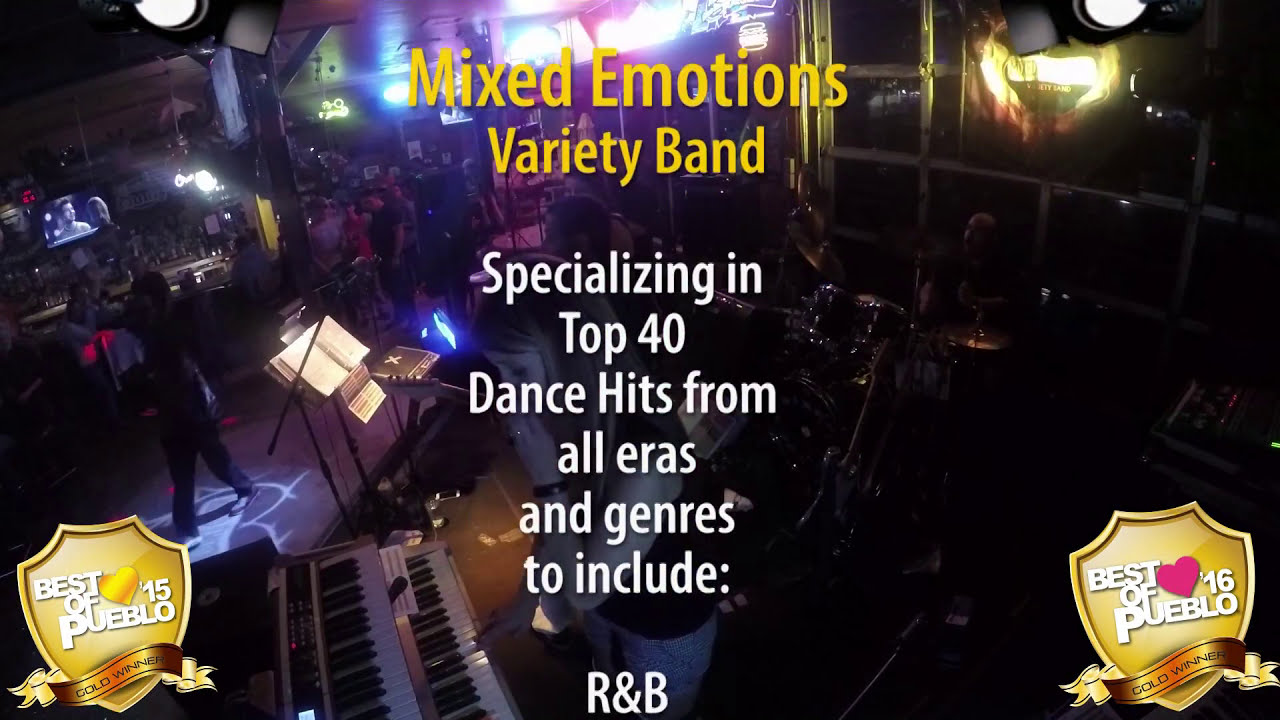The image is a detailed photograph taken inside a dimly lit bar, possibly a sports bar, showing a live performance by a band. The stage is set with various musical instruments, including a double-sided keyboard played by a lady on the left, a drum set, and a guitarist standing behind her. The scene captures the typical ambiance of a lively bar with people standing around, a small TV visible in the background, and shelves lined with liquor bottles.

Above the band, the text "Mixed Emotions Variety Band" is prominently displayed in large yellow letters. Below that, in white lettering, the caption reads, "Specializing in Top 40 dance hits from all eras and genres to include R&B." This indicates the band's diverse musical repertoire.

On the bottom corners of the image, there are two gold shield logos with "Gold Winner" banners. The left shield bears the text "Best of Pueblo 15" and has a gold heart, signifying an award from 2015. The right shield reads "Best of Pueblo 16" with a pink heart, indicating a similar accolade from 2016. The spotlight in the upper right corner and additional lights above the stage accentuate the band's performance area, adding to the vibrant atmosphere of the photograph.